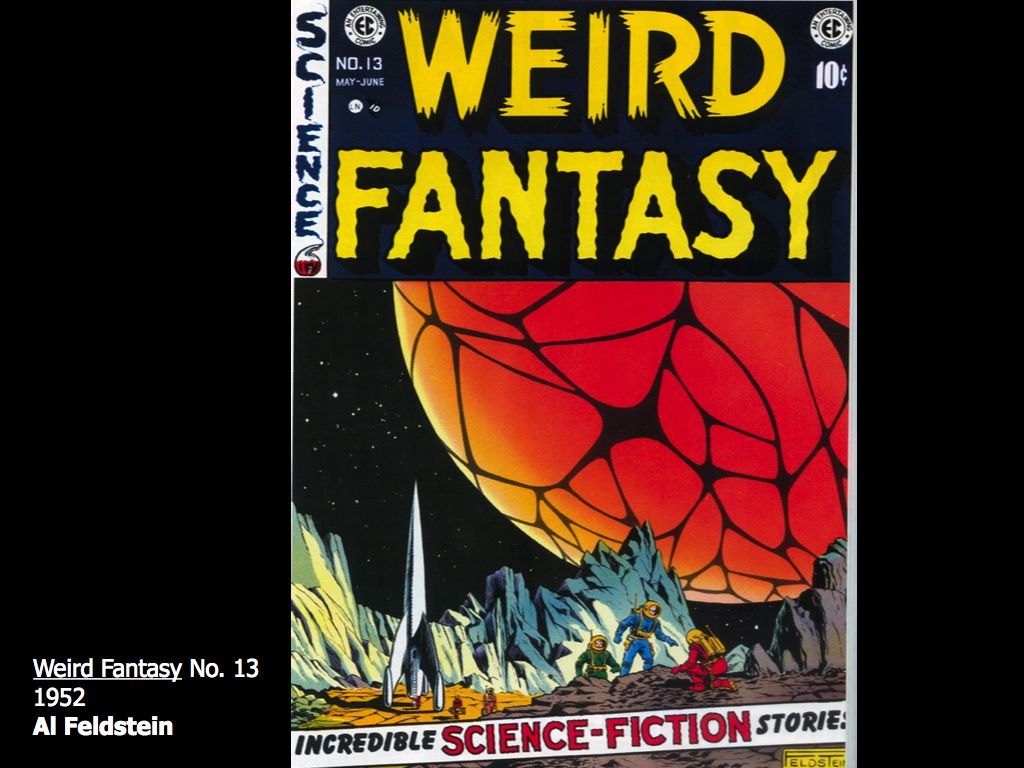This image depicts the cover of a comic book titled "Weird Fantasy." The title spans two lines at the top, with "Weird" on the first line and "Fantasy" on the second, both in large, striking yellow letters against a dark backdrop. The word "Fantasy" has wavy outlines that add a dynamic effect. Vertically on the far left, "Science" is printed in blue letters. Below this, at the bottom of the cover, the phrase "Incredible Science Fiction Stories" is prominently displayed.

The artwork features a mesmerizing alien landscape. Dominating the center of the cover is a vibrant, reddish-orange planet with a web-like texture, floating against a star-speckled space background. In the foreground, three astronauts in spacesuits are seen navigating a brown rocky terrain. To their left, a sleek rocket ship stands ready, framed by a distant mountain range. The artistic details combine to portray an otherworldly scene brimming with adventure and mystery. Along the bottom left edge of the comic book cover, it is noted as "Weird Fantasy No. 13, 1952," attributed to Al Feldstein.